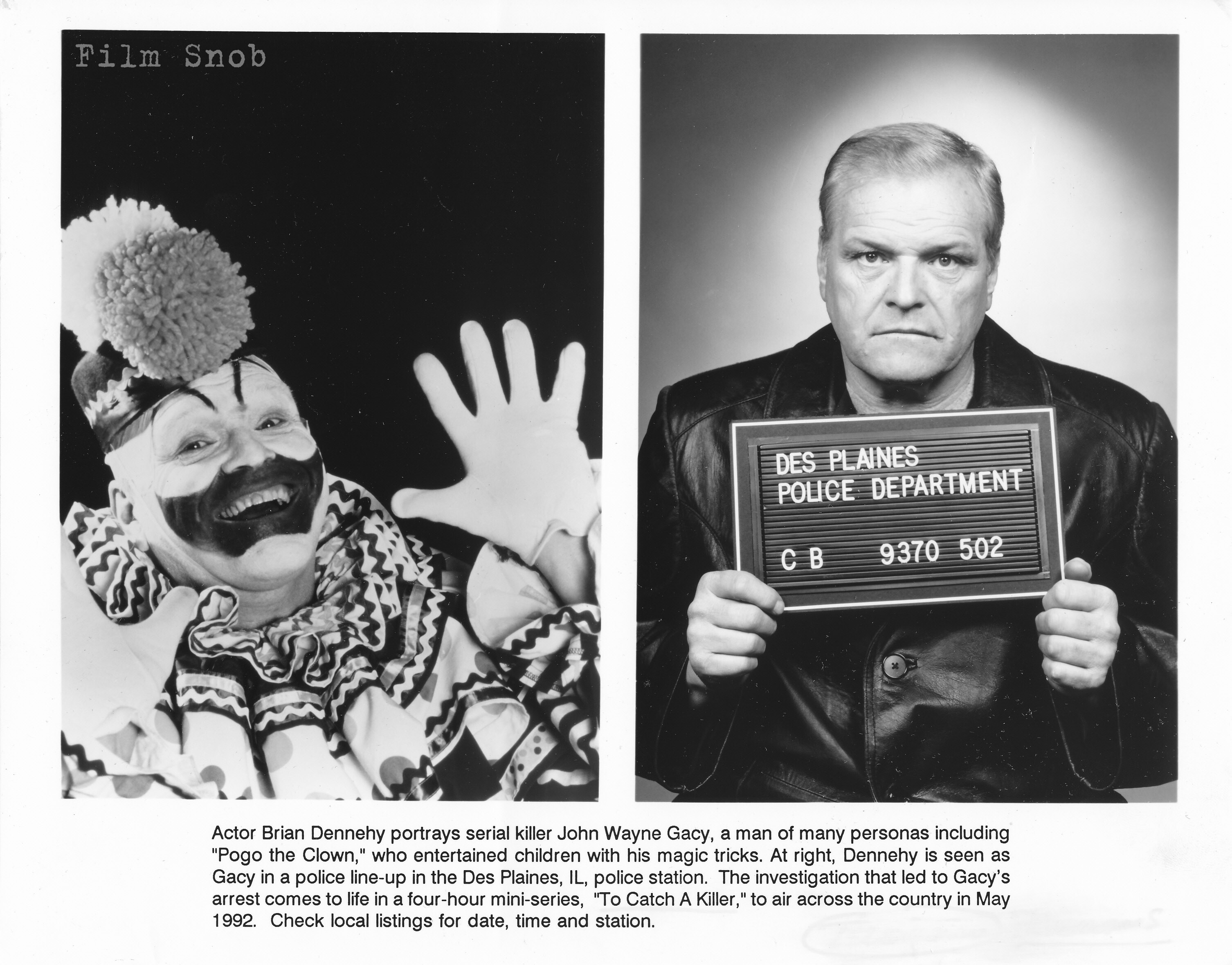This black and white image features two distinct sections placed side by side, clearly showcasing different aspects of a gripping upcoming miniseries. On the left, we see actor Brian Dennehy fully transformed into the infamous serial killer John Wayne Gacy's clown persona, Pogo the Clown. Gacy, famously known for entertaining children with his magic tricks while concealing his darker side, is depicted in full clown makeup including a hat and suit. On the right, Dennehy is shown in a mugshot-style photo, holding a placard from the Des Moines Police Department, dressed in a black leather coat, and appearing significantly older, around 55 years of age.

At the bottom of the image, text informs viewers that Dennehy portrays John Wayne Gacy, a man of many personas, in a four-hour miniseries titled "To Catch a Killer," which brings to life the investigation leading to Gacy's arrest. The series is set to air across the country in May 1992, with viewers advised to check local listings for specific dates, times, and stations. The precise details and layout suggest this image functions as an advertisement for the upcoming series. The image, dominated by shades of black, white, and grey, effectively highlights the stark contrast between Gacy's public and private personas.